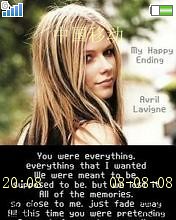This is an image likely from a music cover or screenshot of an electronic device featuring Avril Lavigne. The scene is outdoors with blurred trees in the background. Avril Lavigne is pictured in the center, looking over her shoulder with a slight smile. The screen shows a full signal bar on the top left and a battery icon on the top right, indicating more than half charge. Beside Avril's picture, the text reads "My Happy Ending, Avril Lavigne." Below her image, within a black rectangle, are the lyrics: "You were everything, everything that I wanted. We were meant to be, supposed to be, but we lost it. All of the memories so close to me just fade away. This time, you were pretending." A timestamp with yellow digits "2008 08 08" appears over the text.